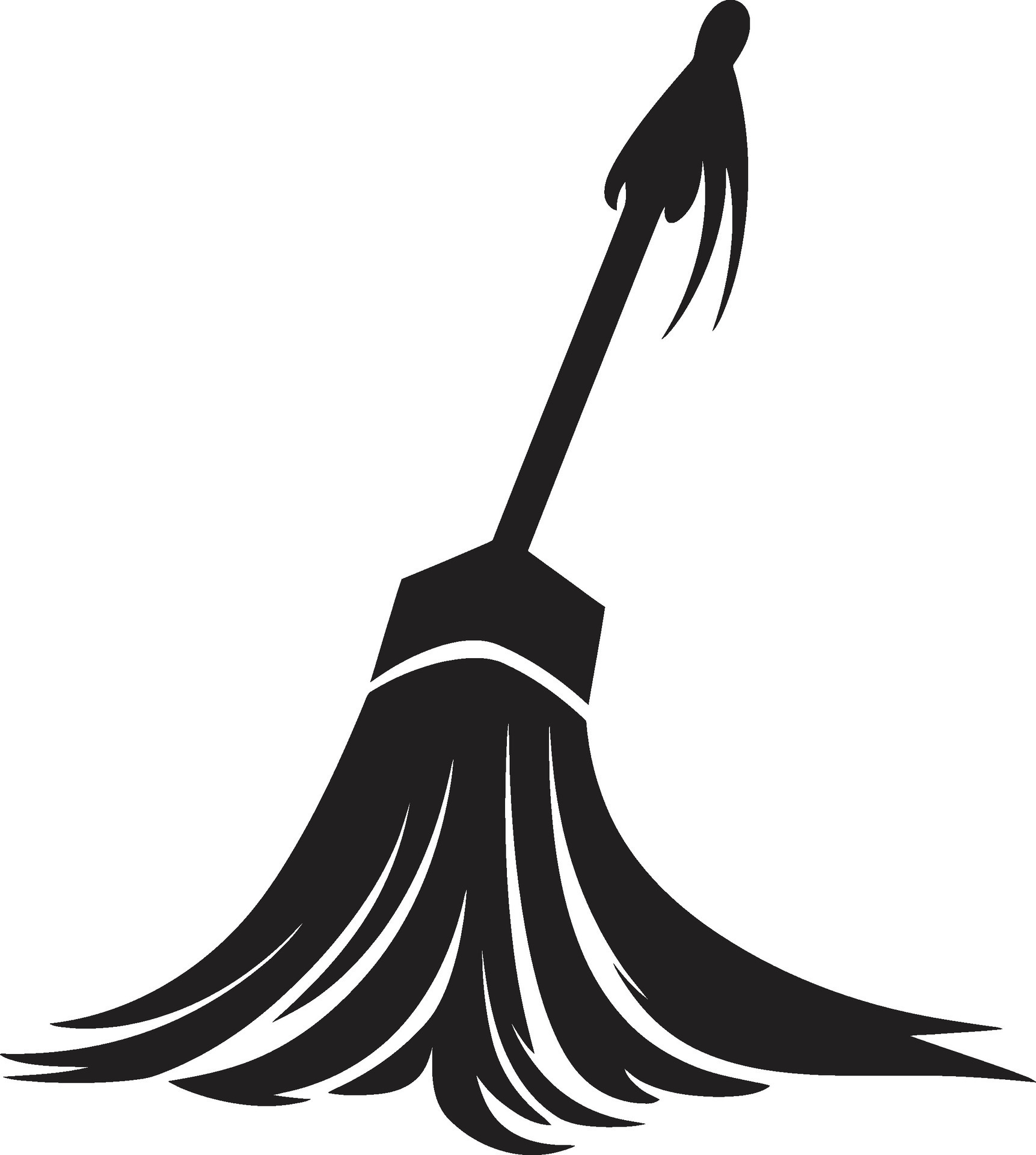The image depicts a digitally rendered, black silhouette of a cleaning tool set against a white background. The tool features a short, narrow handle about 2 feet long, with a band near its end. The head of the tool, which is wide and thick, strongly resembles a broom or feather duster. Its material appears to be spread out, possibly pressed against the floor, with a white line toward the top adding some contrast. Adding an artistic twist, the top of the handle includes an abstract shape reminiscent of a human form with tusk-like projections, enhancing the tribal tattoo-like appearance of the overall design.